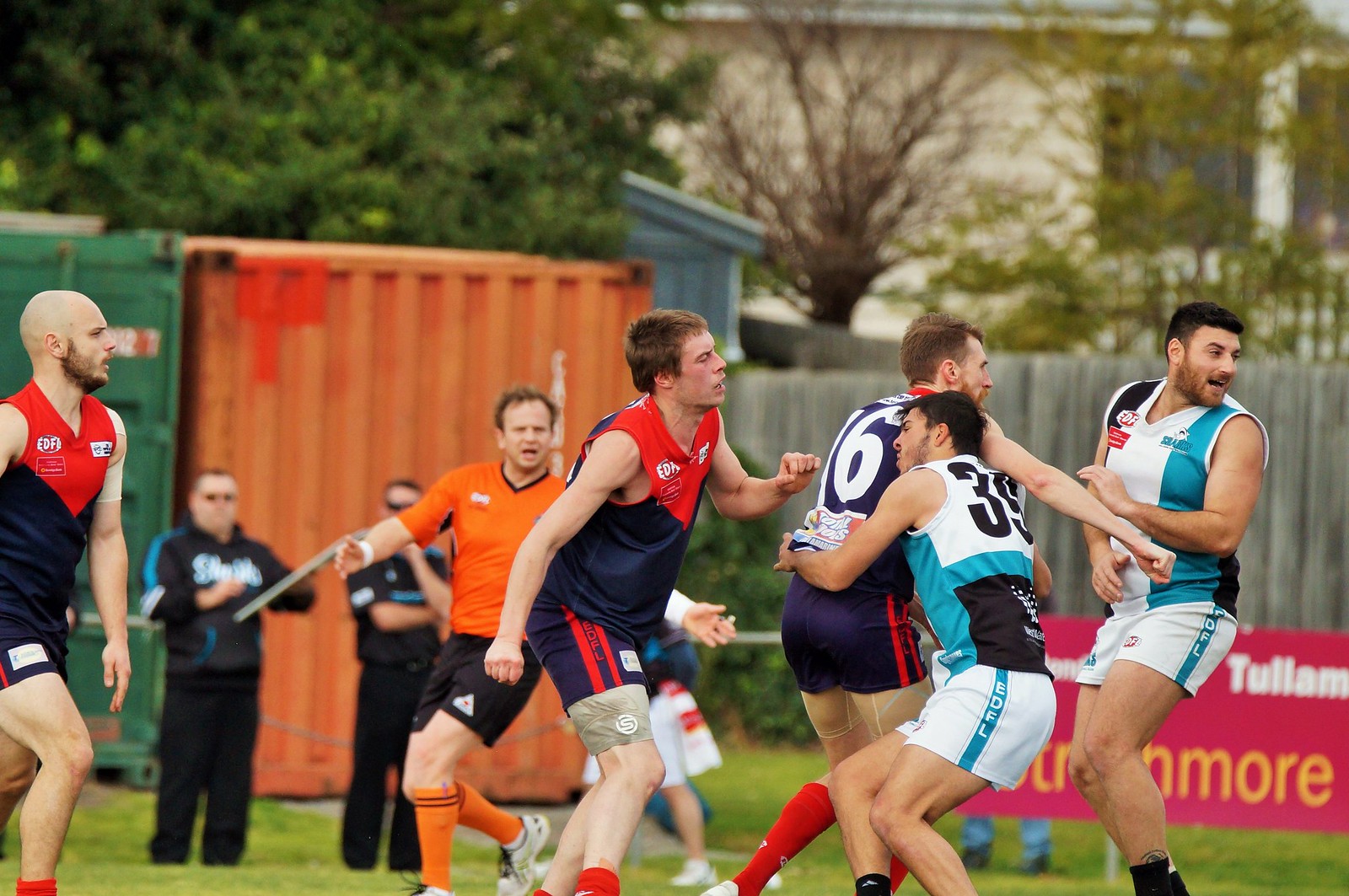In this image, a group of male soccer players are engaged in what appears to be a casual soccer match on a field, evidenced by the absence of a large stadium or substantial audience. There are two teams, distinguishable by their uniforms: one team wears white and teal tops with black accents and white shorts featuring teal stripes with the text "EDFL" inscribed, while the other team sports dark blue shirts with red shoulder accents and blue shorts. The player in the dark blue jersey, marked with the number 6, is facing away from the camera, seemingly being tackled by another player in the white and teal uniform. Another player in the white and teal shirt, also facing left but looking back towards the right, is seen alongside another player in blue and red on the left side of the image. 

In the far background, a bald man and another individual, possibly a referee given his distinctive orange shirt with a v-neck and black shorts, stand near the edge of the field. Also visible on the sidelines are two individuals with their hands folded across their chests, next to conspicuous large industrial containers, one orange and one green, suggesting a non-professional setting. Overall, the scene captures a spirited moment of competition amidst a modest and informal environment.